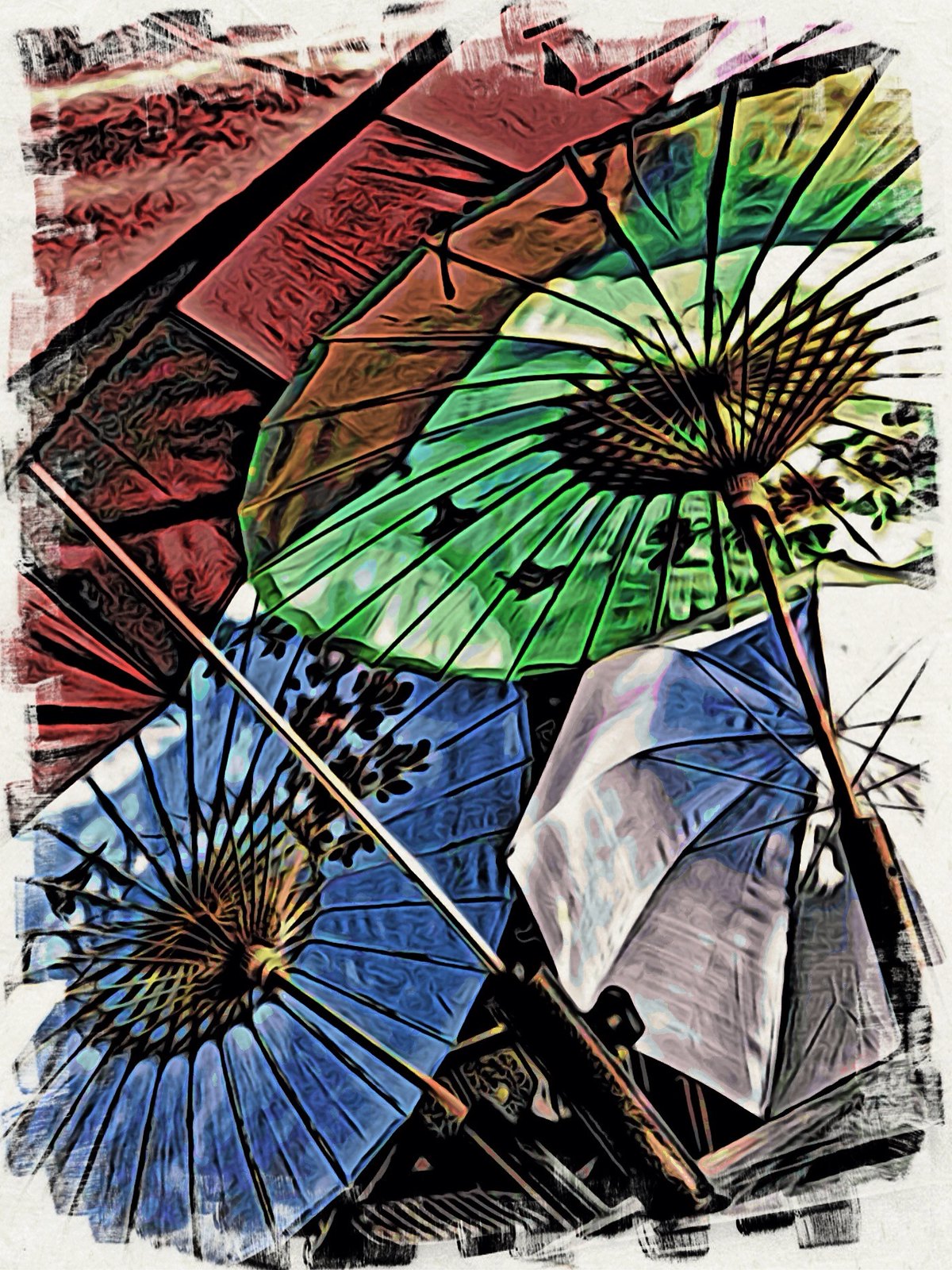This is a vibrant illustration, possibly a computer-created artwork, depicting the underside of several colorful umbrellas viewed from below. The image showcases intricately detailed umbrella spokes, suggesting an abstract design. Dominating the top right portion of the illustration is a green and white umbrella with red edges and a bronze handle; its underside reveals a decorative black pattern against a translucent background. In the bottom left corner, a similar umbrella appears, featuring blue with white edging and also supported by a bronze handle. At the bottom right, a traditional white umbrella with a blue center and a metallic handle stands out. The top left of the image introduces a red background that might represent either another umbrella or the eave of a roof, adding to the complexity of the illustration. The composition is set against a backdrop of red that might contain further patterns. The overall aesthetic is enhanced by brushstroke-like textures around the edges, contributing to the print’s abstract and pleasing effect.